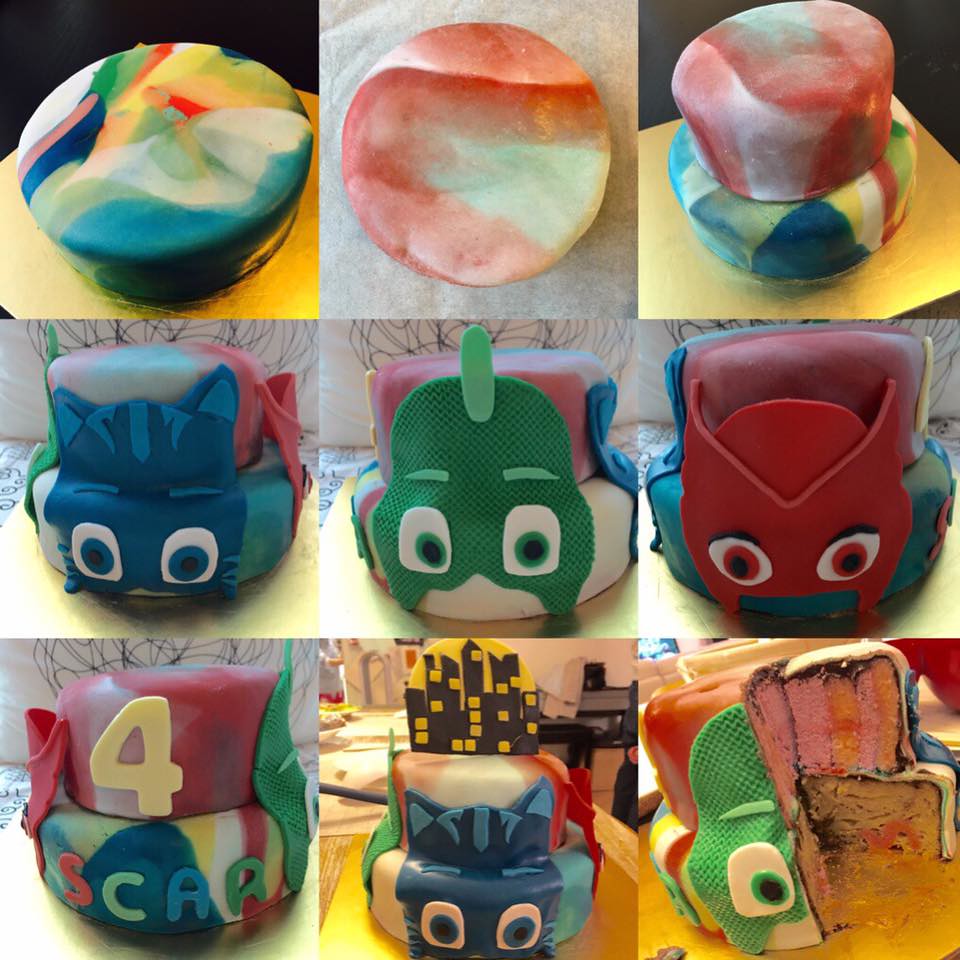This collage of nine images presents a detailed and vibrant overview of a children's birthday cake inspired by PJ Masks, organized in a 3x3 grid format. The upper-left image initiates the series with a colorful, circular base layer of the cake, adorned in rainbow-swirl fondant featuring hues of white, yellow, blue, and pink, and displayed on a gold pedestal. The top-center image offers a top-down perspective of the smaller, upper layer, revealing a fondant design swirled in peach and white. In the top-right image, these base and upper layers are stacked, combining the multicolored and the peach-white layers into a single masterpiece.

Moving to the middle row, the first image showcases a blue PJ Masks-inspired cat figurine with white googly eyes, blue whiskers, eyebrows, ear details, and markings attached to the cake's side. Next to it, the center image displays a green-faced character with textured details including white eyes, green irises, and black pupils. The image on the right in this row features a red-faced character with football-shaped eyes, red irises, and black pupils, intricately finished with black eyeliner.

The bottom row starts with the left image highlighting the cake with a yellow number "4" on the top layer and the word "SCAR" spelled in multicolored letters on the lower layer (S in red, C in green, A in blue, R in dark green). The center image switches to the blue PJ Masks cat, complemented by a city skyline in black silhouetted against a yellow background, indicating a night scene. The final image in the bottom-right corner reveals the cake's internal structure, showing that it is not clay but a cake prepared for the celebration. The green character has been partially sliced, revealing pink layers in the upper tier and vanilla layers in the lower tier, demonstrating the cake's edible artistry.